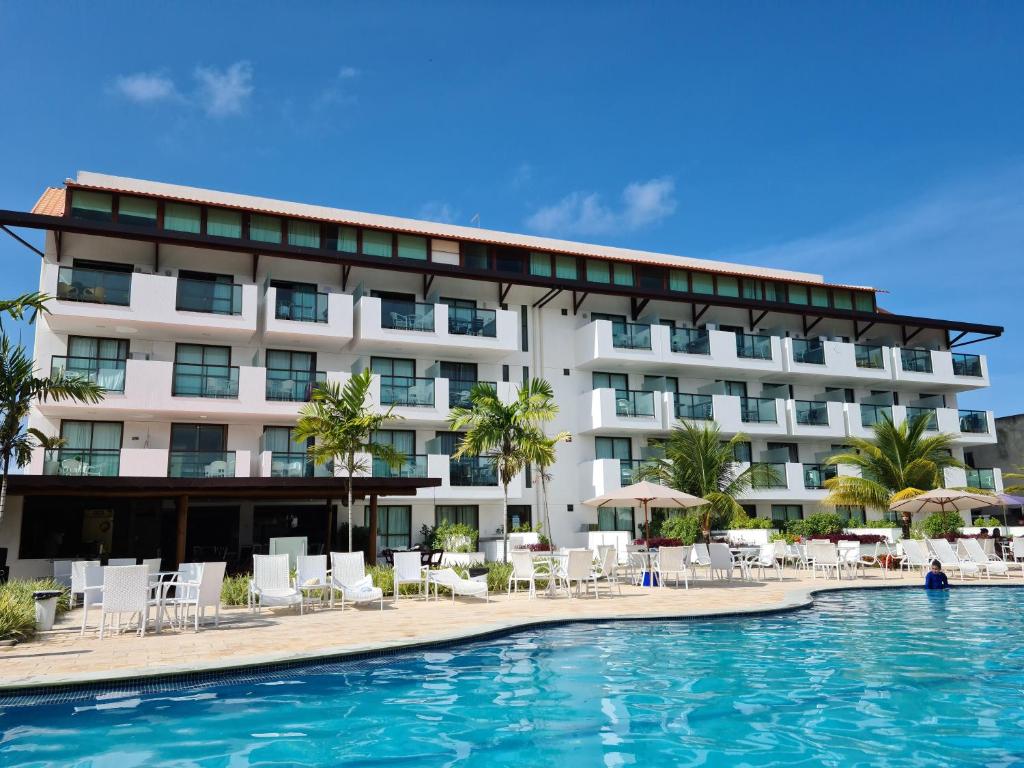This image showcases an exterior view of a large, modern tropical resort, predominantly white with brown trimmings. The resort’s four-story structure is adorned with numerous balconies, all overlooking a pristine, crystal blue pool in the foreground. The pool area is surrounded by white beach chairs and tables, some with umbrellas providing shade, arranged on the concrete sidewalk. Palm trees are interspersed around the pool, enhancing the tropical ambiance. A woman, wearing a blue rash guard, is sitting in the pool on the right side. The sky above is a brilliant blue with wispy clouds, adding to the serene and picturesque setting.